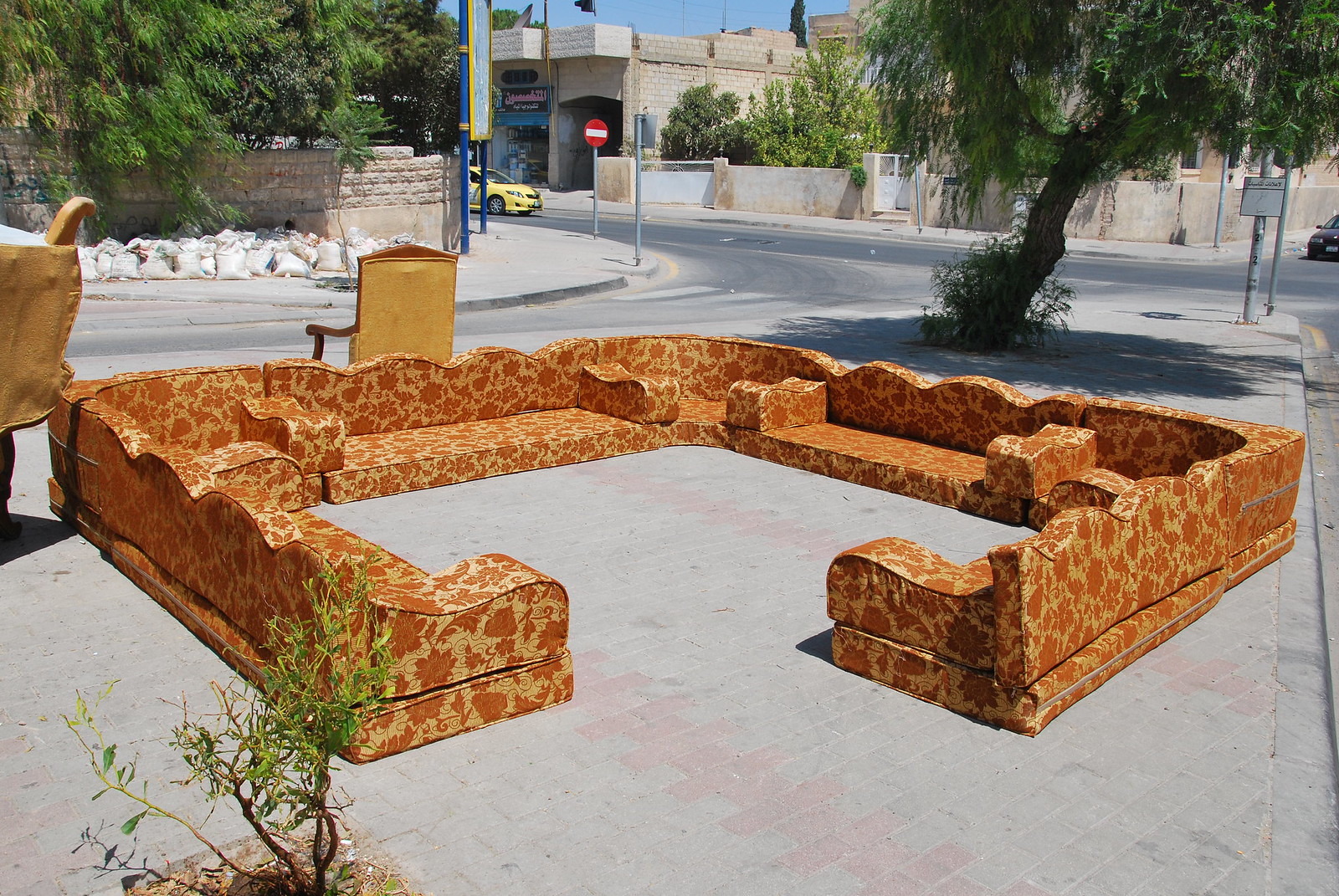This detailed color photo captures a striking outdoor installation of a sectional sofa arranged in a nearly complete square, with one corner open. The sectional is covered in a shiny gold material with orange or rust-colored floral embroidery. The sofa is placed directly on a pavement, which appears to be interlocking pavers, situated on a brick median between two streets in a populated area. There are five armrests spread across the seven sections of the sofa. 

Complementing the sectional is at least one matching chair, though only the chair’s back is visible. The scene also includes a small potted tree in a pavement cutout and a larger shade tree nearby, with branches hanging down and some weeds around the base. Across the median, lined garbage bags and a green tree can be seen, along with a yellow cab approaching. The intersection beyond is a busy five-way junction, surrounded by tan brick buildings. The clear day and various street signs add to the urban ambiance of this unique outdoor setting.